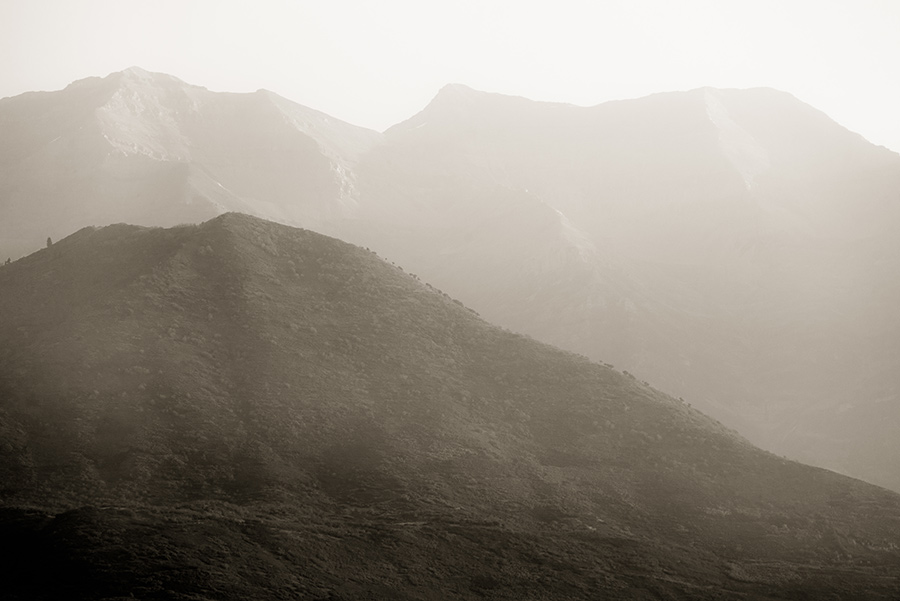In this rectangular landscape photograph, the scene is dominated by an eerie, gray, and hazy atmosphere with muted browns and grays accentuating the somber mood. In the foreground, a prominent mountaintop occupies the left half of the image, covering roughly 50% of the photograph and gradually sloping downwards to the right. The visible portion of this mountain is primarily dark gray with subtle hints of muted green, indicating sparse forestry. Vaguely in the distance on this mountain, a line of what might be cattle or horses can be faintly seen either ascending or descending.

The background showcases a series of jagged, rocky mountains shrouded in mist, making the details indistinct. These distant mountains extend horizontally across the image, occupying about 75% of the frame, with sharp peaks rising and falling, creating a dramatic contrast with the smoother hill in the foreground. The upper portion of the photograph is filled with a featureless, white sky, free of clouds, contributing to the overall foggy and ethereal quality of the landscape.